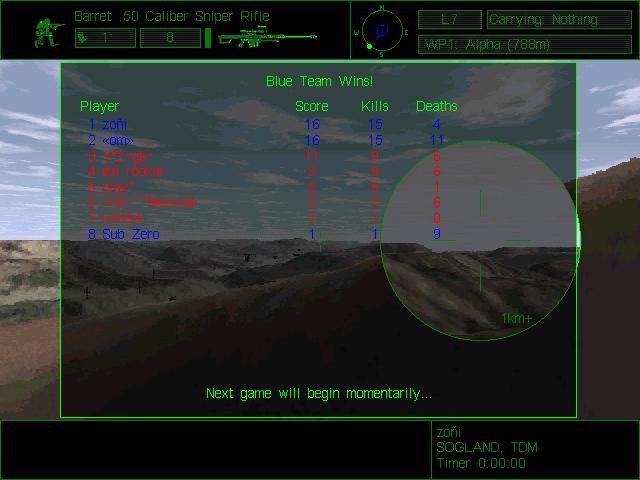This vibrant color image captures a computer screen displaying a dynamic gaming interface. The main focus is a semi-transparent control screen, centrally overlaid on a vivid desert landscape. The background showcases a stunning blue sky dotted with clouds, foothills adorned with sparse foliage to the left, and a rugged, brown terrain towards the right.

At the top of the interface, a black band is filled with various green controls and an infographic of a gun or rifle, though the specific writing is not legible. Dominating the central square of the control screen, bright green text announces, "Blue Team Wins." Below this declaration, a detailed table presents players' scores, kills, and deaths, segmented into blue and red categories. Further down, another green notification reads, "Next game will begin momentarily."

Across the bottom edge and right-hand corner, additional black bands frame the interface, containing more faint green text in the lower right corner, which remains unreadable. This intricate interface reflects the excitement and competitive spirit of the gaming environment.